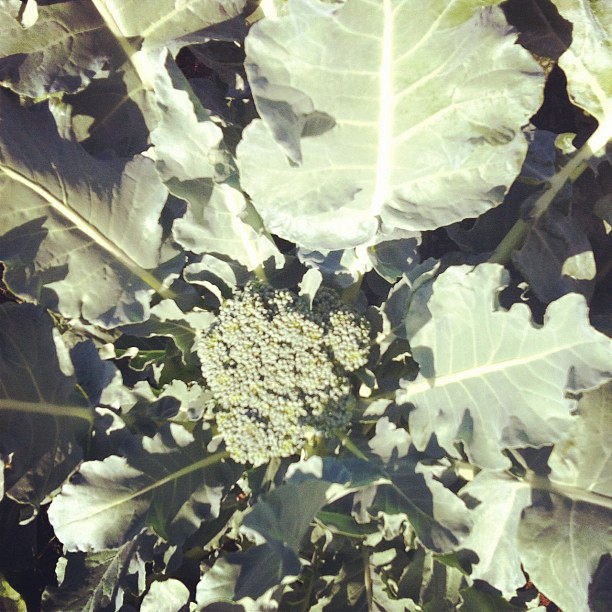This image showcases a close-up of a broccoli plant nestled among dense foliage. The small head of broccoli, which may not be fully matured, takes center stage, surrounded by five prominent large leaves exhibiting a rich green hue. Each leaf displays a central vein with branching yellowish-white lines extending outwards. Additional smaller leaves envelop the plant, contributing to the lush greenery that covers nearly the entire frame. The interplay of light and shadow suggests the sun is nearly overhead, casting a small shadow from the broccoli onto the surrounding leaves, while other parts of the vegetation show varied shades of green due to the sunlight hitting them at different angles. The dense foliage indicates either a densely planted farm or a thriving garden, with no soil visible beneath the verdant mass.